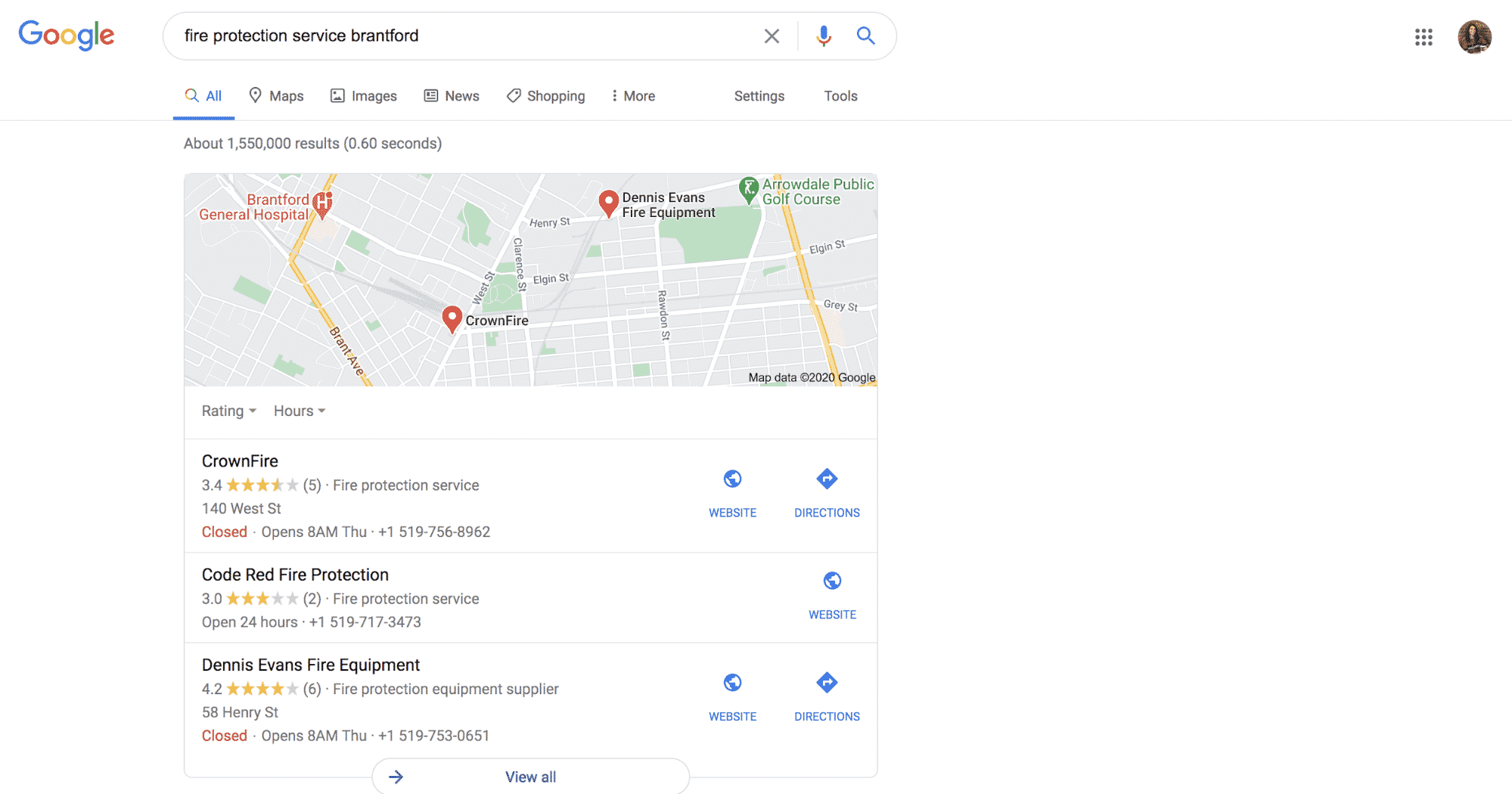This color screenshot from Google features its iconic logo in the top left corner, with "Google" spelled out in multi-colored letters: a blue 'G', a red 'O', a yellow 'O', a blue 'G', a green 'L', and a red 'E'. Below the logo is the search bar, displaying the query: "Fire Protection Service Brantford".

An inset map highlights various locations marked in Brantford, including Brantford General Hospital, Crown Fire, Dennis Evans Fire Equipment, and Arodale Public Golf Course. Notable businesses listed are:

1. **Crown Fire**:
    - Rating: 3.4 stars out of 5 based on 5 ratings
    - Type: Fire Protection Service
    - Address: 140 West Street
    - Status: Closed, opens at 8 a.m. on Thursday
    - Contact: 1-519-756-8962
    - Features: Website, directions

2. **Code Red Fire Protection**:
    - Rating: 3.0 stars based on 2 ratings
    - Type: Fire Protection Service
    - Status: Open 24 hours
    - Contact: 1-519-717-3473
    - Features: Website

3. **Dennis Evans Fire Equipment**:
    - Rating: 4.2 stars out of 5 based on 6 ratings
    - Type: Fire Protection Equipment Supplier
    - Address: 58 Henry Street
    - Status: Closed, opens at 8 a.m. on Thursday
    - Contact: 1-519-753-0651
    - Features: Website, directions

At the bottom of the screen, there's an option labeled "View All" for more search results or information. The map data is credited to "Mapdata 2020 Google".